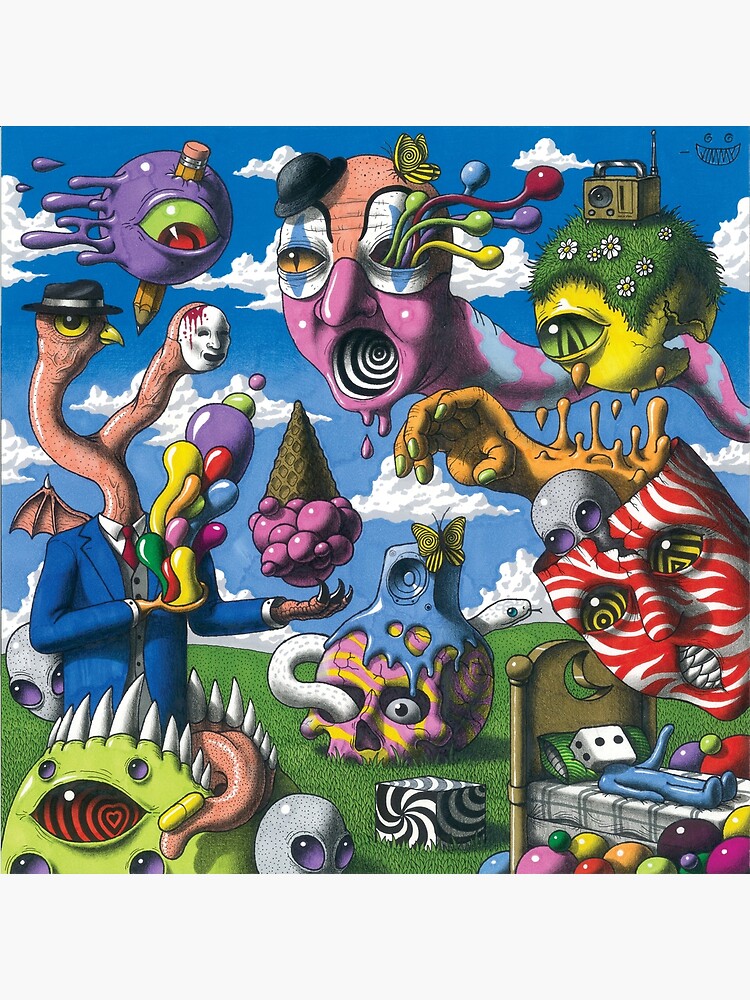In this psychedelic, surreal artwork, multiple elements create a mesmerizing and intricate scene. The background features a brilliant blue sky dotted with fluffy white clouds and a vibrant green field. A potential signature of the artist, resembling a monstrous face, is located in the top right corner. 

In the top left, a purple floating eyeball, pierced by a pencil, captures immediate attention. The eyeball is vividly white with red details. Just to its right, a whimsical floating worm adorned in clown makeup appears. The worm's body is striped in pink and blue zig-zags and it wears a top hat tilted jauntily atop its head. From one eye socket, an ambiguous stream of either sperm or balloons emerges, while its mouth is illustrated as a hypnotic spiral.

Further right, another floating eyeball colored yellow with a green iris stands out. This eyeball has grass with daisies growing on it, and atop it rests a small radio. At the center of the image, a peculiar two-headed gentleman commands attention. One of his hands, equipped with claws, holds an ice cream cone upside down. The other hand, transformed into a spoon, drips with rainbow-colored blobs. Both of the gentleman's heads exhibit a warm demeanor; one wears a bloody mask, while the other features a bird's head capped with a top hat. This fantastical creature is further adorned with bat wings.

Moving towards the middle, a pink and yellow skull with a white snake winding through it presents a haunting yet captivating focal point. On the skull, a melting blue speaker and a delicate yellow butterfly add layers of texture and color. On the right, a red and white striped floating mask conceals an alien figure peeking out. The alien extends a yellow monstrous hand with green fingernails.

Towards the bottom of the image, a collection of otherworldly creatures completes the scene. These include a green monster with white spikes on its head and a blue humanoid figure with a die for a head, resting on a bed surrounded by balloons. This highly intricate and artistically vibrant image distinctly stands out as a hallmark of psychedelic art.